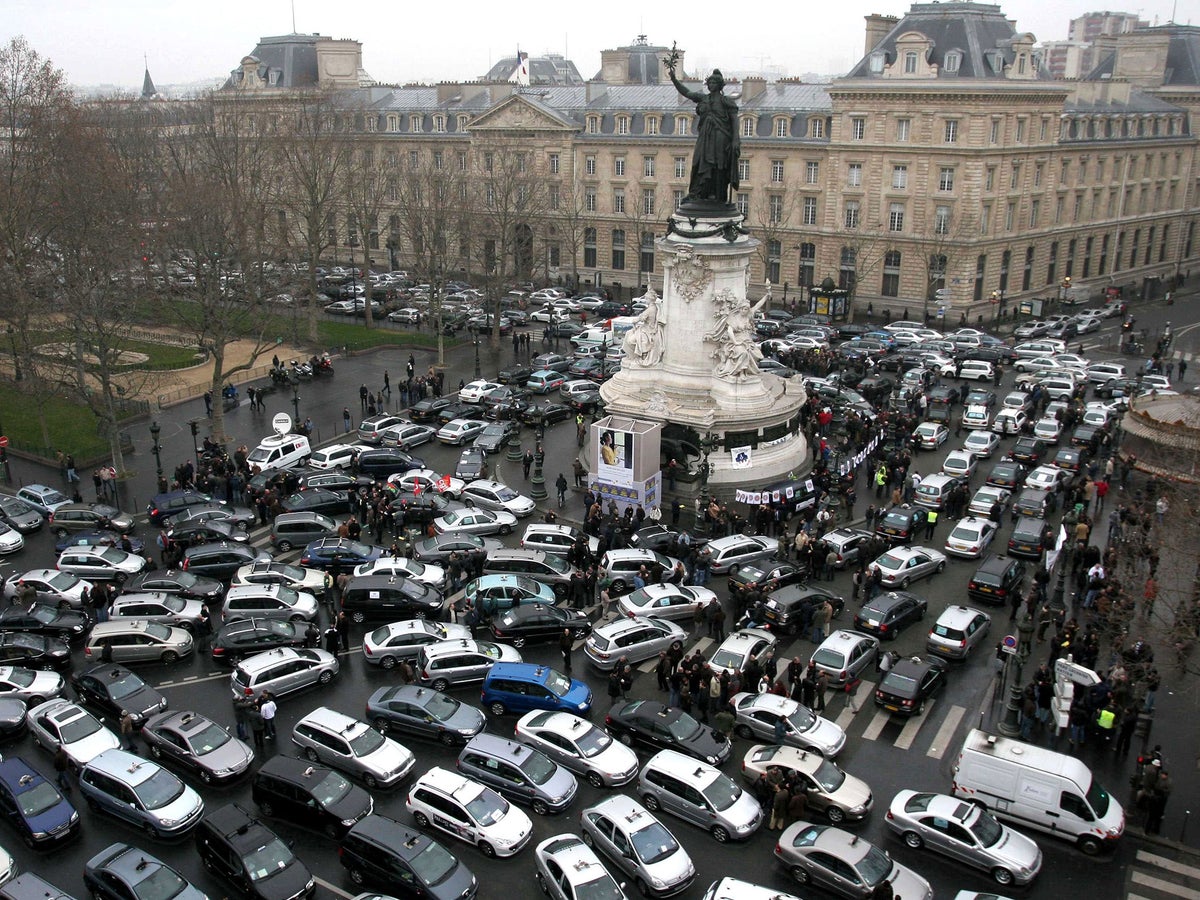The image depicts a bustling urban scene, likely in Paris, showing a significant traffic jam around a large circular monument. The background is dominated by a colossal, landmark stone building that spans multiple blocks and features flags, suggesting it is an official or historical structure. In the foreground, the traffic converges around a grand white stone pedestal supporting a black metal statue, possibly of a woman, raising its right arm into the air. This monument acts as the center of a roundabout, with numerous cars, possibly taxis and hired rides, moving haphazardly around it without defined lanes. The sheer volume of vehicles, showing a mix of black and silver, appears indicative of a protest or strike, contributing to the standstill traffic. The image captures the essence of a dynamic and congested city street, characteristic of Parisian life.